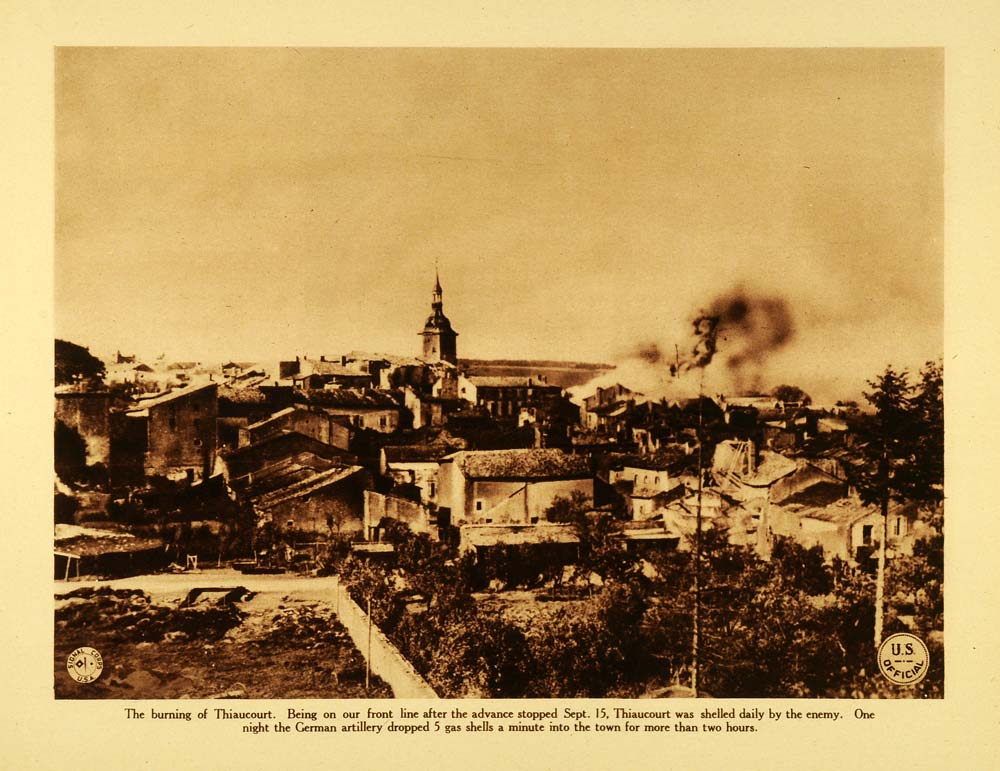This is a vintage black-and-white photograph of the bombed city of Theochort, Germany, printed on yellowing paper. The scene captures the aftermath of a relentless bombardment by German artillery. Smoke, indicative of a recent explosion, billows from the upper right-hand side of the image, looming over the town. The city is mostly in ruins, with dilapidated buildings dominating the background and scattered rubble and dirt in the foreground. A few relatively intact buildings stand precariously in the middle foreground. The tallest structure, a steepled building, possibly a church, rises prominently in the background. The photo's caption explains the context: "The burning of Theochort, being on our front line after the advance stopped September 13. Theochort was shelled daily by the enemy. One night, the German artillery dropped five gas shells a minute onto the town for more than two hours." This U.S. Army photograph, stamped "U.S. official" in the bottom right corner, starkly illustrates the devastation wrought by continuous enemy shelling.